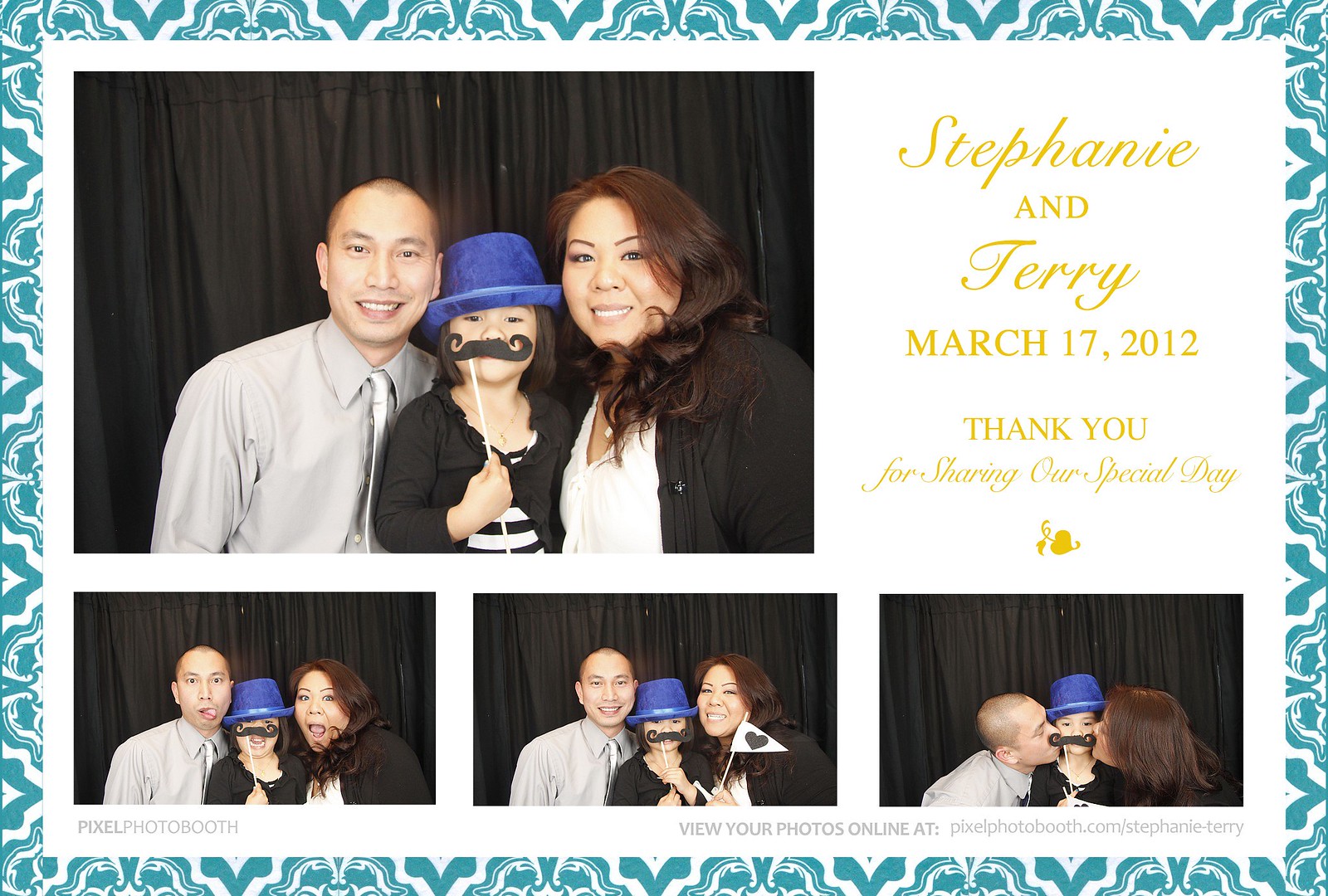The image depicts a thank you card with a bluish border and a white background. At the top left is a large photo booth picture of an Asian couple with their young daughter, who appears to be about five years old. The man, wearing a gray collared shirt and silver tie, and the woman, dressed in a black cardigan over a white shirt, are both smiling at the camera in front of a black curtain backdrop. Between them is their daughter, who is wearing a black sweater over a black and white striped shirt, a blue fedora, and holding a fake mustache on a stick up to her face.

To the right of this large image, in gold lettering, the text reads: "Stephanie and Terry, March 17, 2012. Thank you for sharing our special day." Along the bottom of the card are three smaller photo booth pictures of the same family. In the leftmost photo, they are making silly faces by sticking out their tongues. In the middle photo, they are all smiling, with the mother holding up a small flag featuring a heart. In the rightmost photo, both parents are kissing their daughter on the cheeks, and the daughter still has the fake mustache up to her face in all the photos.